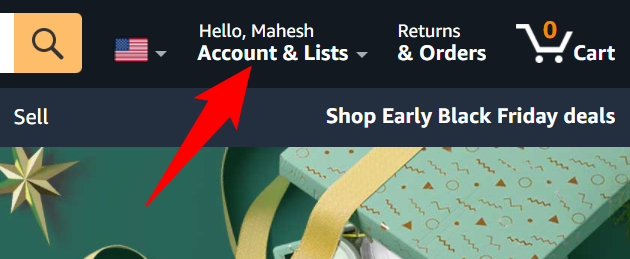This close-up image of an Amazon webpage highlights the "Accounts and Lists" section. Positioned on the right side of the top black navigation bar, the "Accounts and Lists" text appears in bold white font, situated above a greeting that says, "Hello, Mahesh" in white font. A red arrow points directly at this section, emphasizing the current logged-in user and the dropdown menu for account options. To the left, partially visible, are the Search button and part of the search bar, indicating the user’s ability to search for products on the site. Also visible in the top black bar, near the center-left, is the indication that the country selected is the United States. The entire top bar spans from left to right across the image.